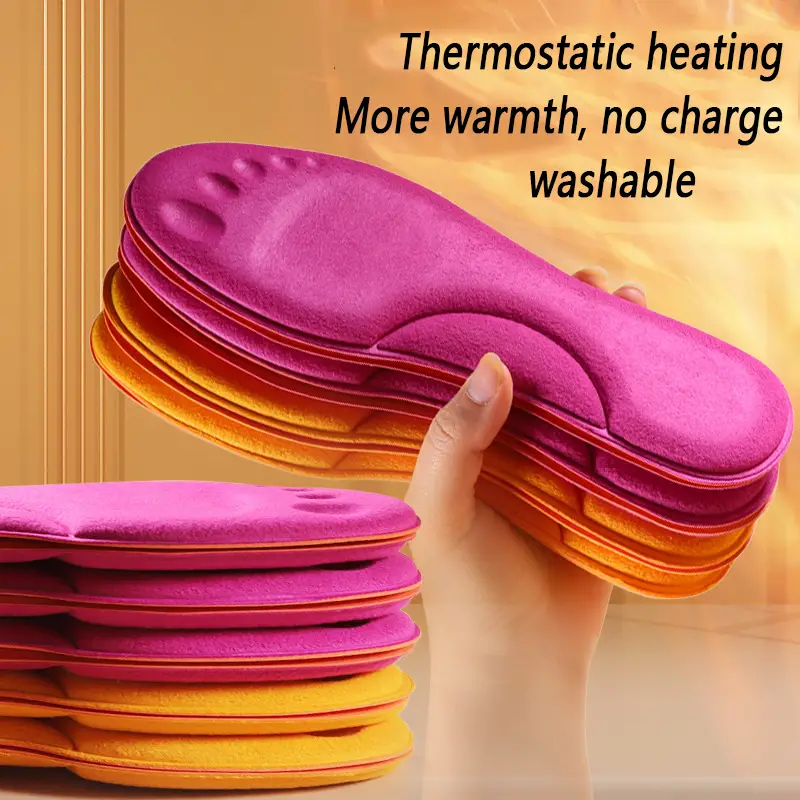The image showcases a product advertisement for thermostatic shoe inserts. The photograph features a hand holding four shoe inserts, two in a vibrant purple and two in bright orange. To the left of the hand, another set of four inserts is arranged vertically, with the top three in purple and the bottom two in orange. The background is a beige color with subtle vertical indents on the top left. In the top right corner of the image, black text reads "thermostatic heating, more warmth, no charge, washable," highlighting the product's key features. This high-quality image effectively captures the details and variations of the shoe inserts, emphasizing their innovative features and vivid colors.